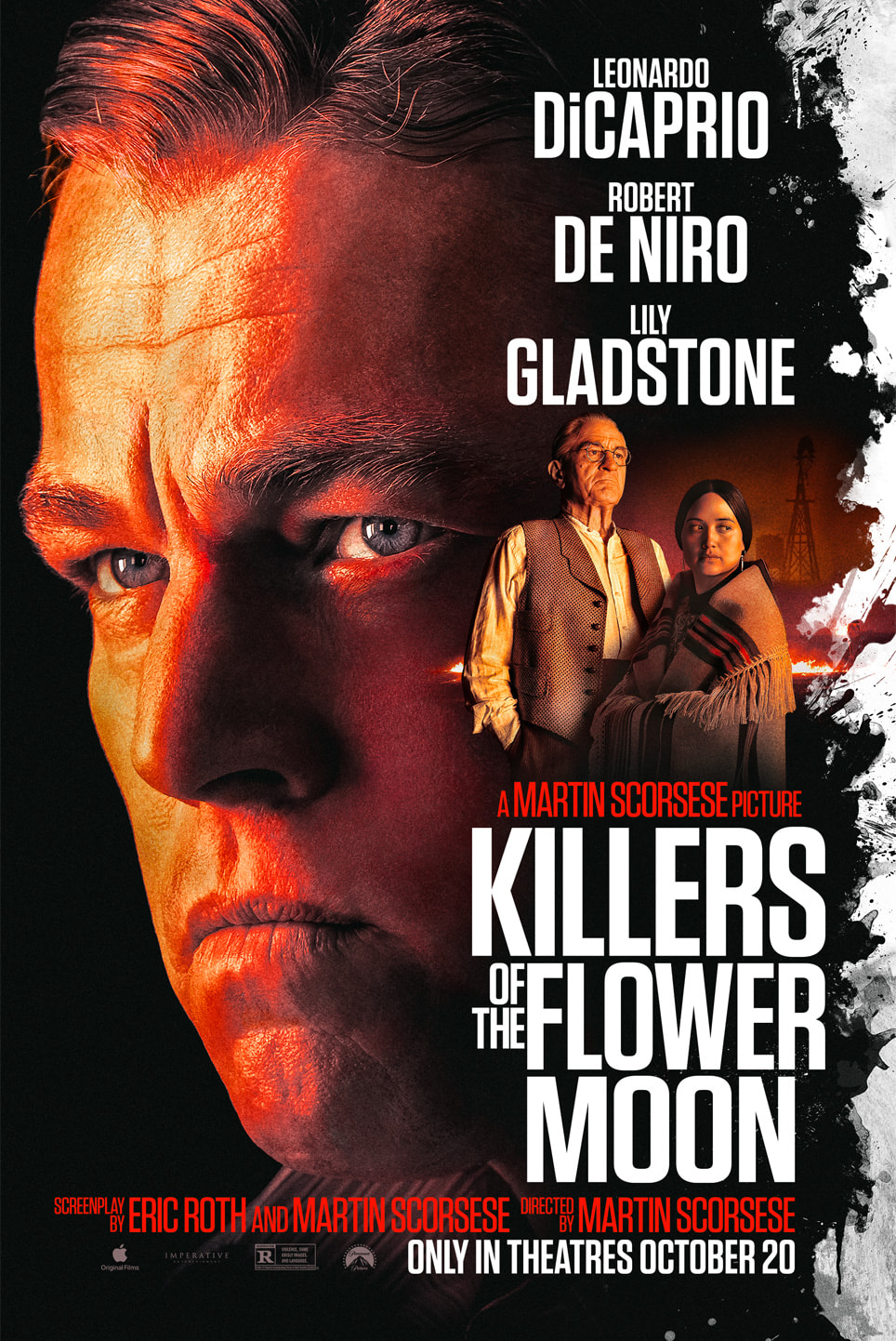The image is a movie poster for "Killers of the Flower Moon," a Martin Scorsese picture. The background is black, and the text is predominantly in all capital letters, with "Martin Scorsese" highlighted in red. At the top, the names of the lead actors—Leonardo DiCaprio, Robert De Niro, and Lily Gladstone—are prominently displayed. 

Leonardo DiCaprio's face is prominently featured on the left side of the poster, turned slightly to the left, exuding a serious expression with his blue eyes and fairly tan skin. His face has an orange glow, and his hair is parted to the side. 

Adjacent to DiCaprio's image are smaller photographs of Robert De Niro and Lily Gladstone. Below their images, text reads "A Martin Scorsese Picture" above the film's title, "Killers of the Flower Moon." The credits at the bottom highlight the screenplay by Eric Roth and Martin Scorsese and specify that the film is directed by Martin Scorsese. The bottom-most text informs viewers that the film will be "Only in Theaters October 20."